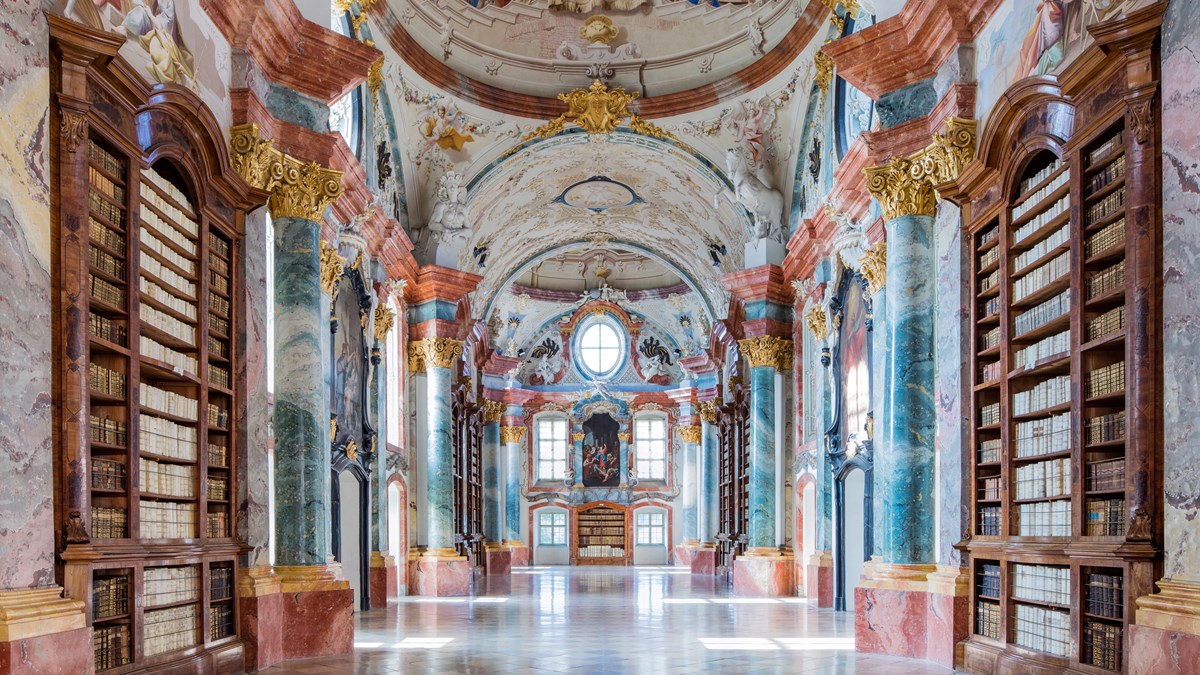In this photograph of a grand and ornate palace hallway, we see a colorful and intricately designed interior that resembles a cathedral. The hallway features a series of tall, inset bookshelves made of polished wood, filled with books, lining both the left and right walls. These bookshelves, divided into three horizontal segments, are set against walls painted in blue and cream colors adorned with detailed designs. The columns throughout the hallway are made of blue and white marble with gold caps, and some have red decorative masonry above them. The floors are shiny and white, reflecting the grandeur of the space.

At the far end of the hallway, there is a painting mounted on the wall, just below a smaller bookshelf. Above the painting is an egg-shaped window that allows natural light to flood into the room. The ceiling is curved and elaborately decorated with gold, blue, and white patterns, adding to the overall opulence. The room is awash with daylight from several windows, highlighting its vibrant and sumptuous decor, making it a splendid example of luxurious palace architecture.